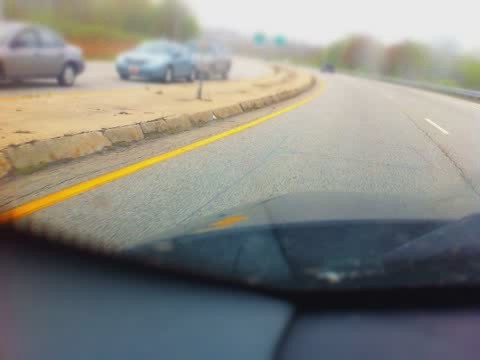This color photograph, despite its low resolution and blurred background, captures the view from the driver's perspective inside a vehicle. The camera is positioned on the dashboard, nestled in the bottom left corner of the windscreen. The dashboard appears as a slim gray strip at the bottom of the image, while the dark blue, almost black, hood of the car stretches out in front. The scene ahead reveals a multi-lane road with a prominent solid yellow line on the left side and intermittent white dashed lines separating the lanes on the right. A tan-colored, raised median strip runs along the center, demarcating the opposite lane of incoming traffic, which features three visible cars: two gray and one turquoise. The road ahead curves slightly to the left, with large green road signs suspended above, their text too blurry to decipher. Flanking the highway, the right side sports a silver guard rail and a mixture of green and brown trees, all set against a hazy gray sky.